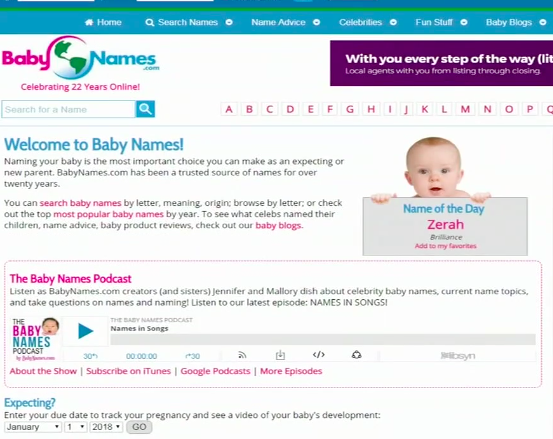The image features a vibrant and interactive baby names website homepage. 

On the left, the word "Babies" is prominently displayed in pink, while on the right, "Names" is highlighted in blue. At the top, six categories are arranged in white text from left to right: Home, Search Names, Name Advice, Celebrities, Fun Stuff, and Baby Blogs. These categories are set against a background with a green line above them and a blue line further above. The main backdrop is white, framed within a purple rectangle.

To the right of the page, a comforting slogan reads, "With you every step of the way," accompanied by a note about local agents assisting from filtering through closing. Below, the alphabet from A to Q is listed in pink text. 

The section titled "Welcome to Baby Names" appears in blue text, just beneath a search bar designed for effortless navigation. Further down are two sentences providing additional details, and to the right, there's an image of a baby's head viewed from the front. 

Highlighted in blue, "Name of the Day" introduces the name "Zera," spelled Z-E-R-A-H, in pink text. Adjacent to this, "Baby Names Podcast" is noted in pink, followed by smaller black text providing more information about the podcast. Below this is another mention of the "Baby Names Podcast," featuring the segment "Names and Songs," along with clickable icons for more details about the show, subscription options on iTunes and Google Podcasts, and access to more episodes, all in pink text.

At the very bottom, the text "Expecting" appears in blue, inviting users to enter their due date to track their pregnancy, with an entry section provided below.